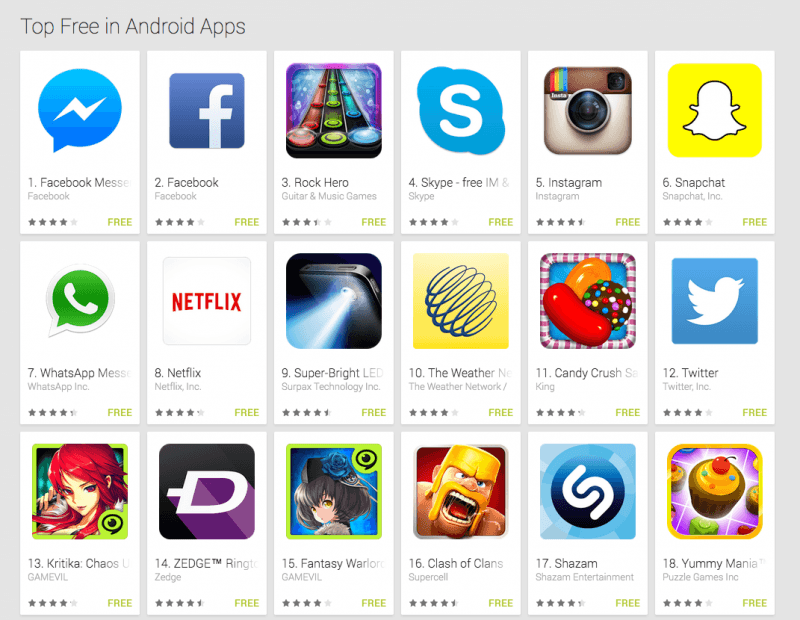The image showcases the top free Android apps available for download, neatly organized into three rows with six apps in each row. Each app tile features the app’s logo, a "Free" label in light green letters at the bottom right corner, and the star rating at the bottom left. The apps displayed are as follows:

**First Row:**
1. Facebook Messenger
2. Facebook
3. Rock Hero
4. Skype
5. Instagram
6. Snapchat

**Second Row:**
7. WhatsApp
8. Netflix
9. Super Bright LED Flashlight
10. The Weather
11. Candy Crush
12. Twitter

**Third Row:**
13. Kritika
14. Zedge
15. Fantasy Warlord
16. Clash of Clans
17. Shazam
18. Yummy Mania

Each app’s logo provides a visual representation of the app, enhancing the ease of recognition for users browsing through these top-rated, free-to-download Android applications.